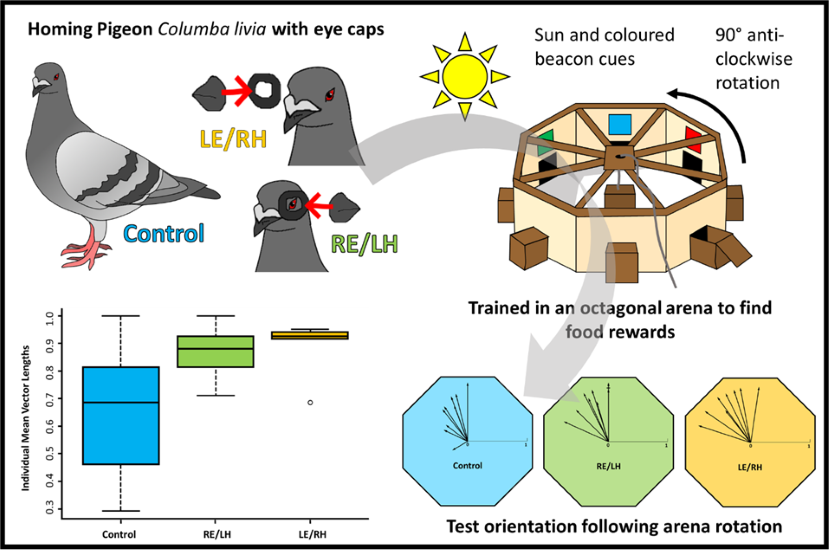The infographic titled "Homing Pigeon, Columbia, Libya" prominently features detailed illustrations and information about homing pigeons. In the top left corner, the title is followed by a yellow sun graphic. To the right of the sun, the text "Sun and Colored Beacon Keys" is noted with notation of "90 degrees anti-clockwise rotation." Below the title, there's an illustrated pigeon labeled "CONTROL" in blue. Beside it, there are close-up images labeled "L-E backslash R-H" and "R-E-L-H," focusing on the pigeon's eye details. 

To the right, an octagonal arena is depicted with visible green, blue, and red segments, indicating a training setup. This is labeled "Trained in an octagonal arena to find food rewards," suggesting pigeons are conditioned within this structure for their homing ability. Below this is a graph titled "Individual Mean Vector Lengths," featuring measured scales from 0.3 to 1.0 with distinct categories for "CONTROL," "R-E-L-H," and "L-E-R-H," represented by corresponding blue, green, and yellow rectangles. 

Further to the right are three octagon graphics labeled "Test orientation following arena rotation," color-coded in blue (control), green (R-E-L-H), and yellow (L-E-R-H), indicating different experimental conditions. Overall, this infographic merges detailed visual and textual elements to explain the training, testing, and behavioral analysis of homing pigeons.